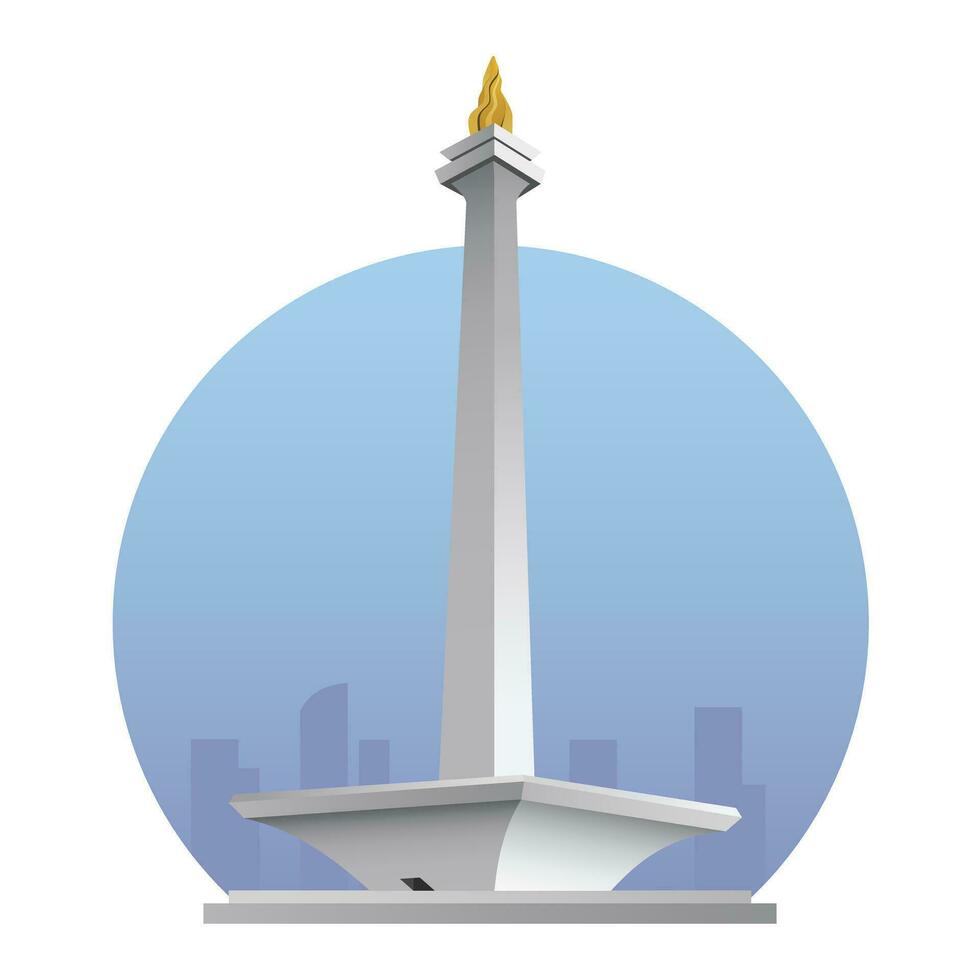This vector illustration depicts a striking scene dominated by a tall, slender pillar crowned with a swirling flame. The pillar, rendered in shades of gray with intricate gradients and shading, supports two rows of small squares near its summit. At the base, it widens into a more substantial platform, which itself rests on a flat, broad foundation, conveying the look and texture of cement.

Above the pillar, the flame spirals in dynamic shades of yellow and golden yellow, drawing the eye upwards. The backdrop features a large, encompassing blue circle that transitions through a gradient from deep to light blue, punctuating the composition. In front of this gradient backdrop, the faint silhouette of a cityscape emerges in dark blue, adding depth and context to the scene. Overall, the illustration artfully combines geometric shapes and gradients to create a serene yet profound visual narrative.